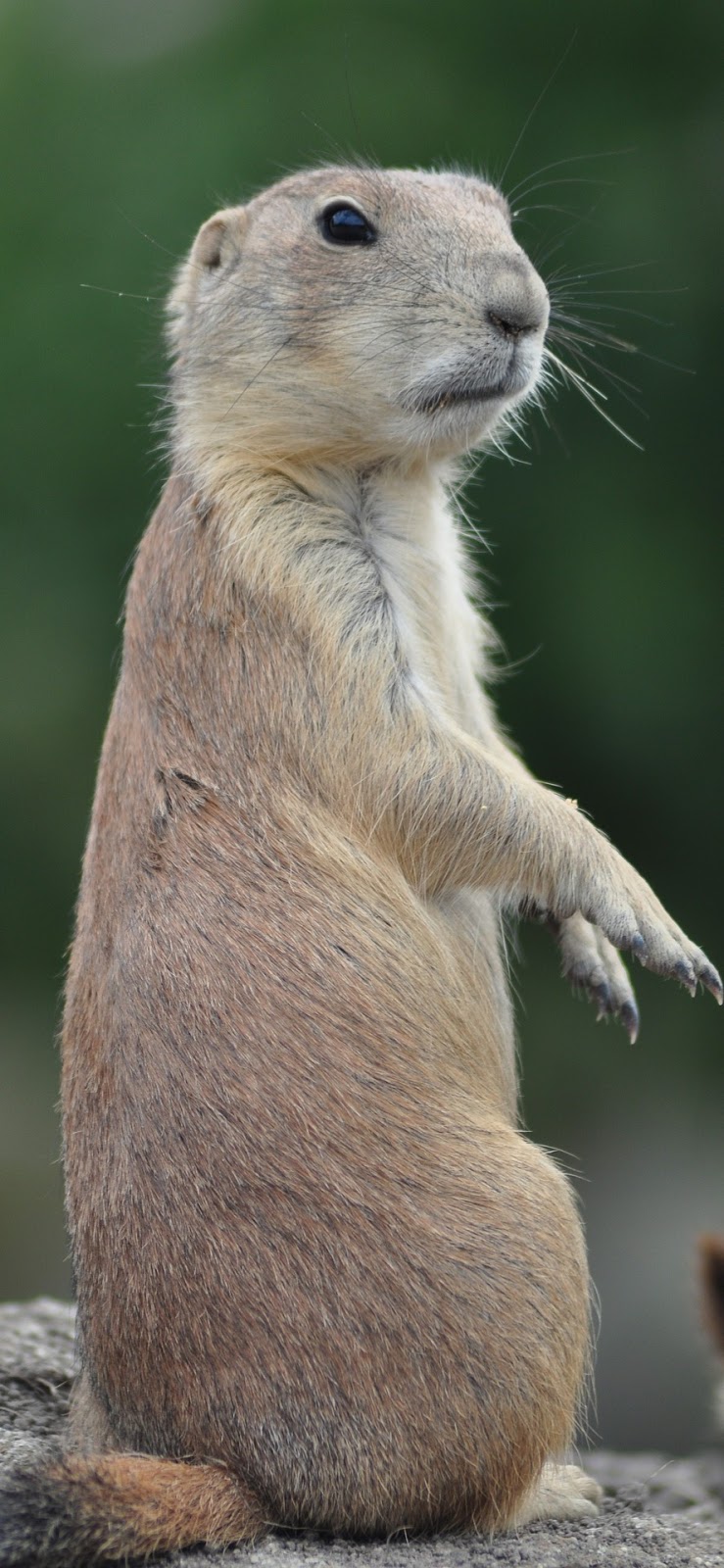This photograph captures a tall, rectangular image dominated by a squirrel standing upright on a gray rock. The squirrel, predominantly brown with patches of white and light gray, occupies nearly the full length of the image, extending from almost the bottom to near the top. Its posture is unusually erect, with its hind legs positioned as if it's partly sitting. The squirrel's head is turned slightly to the right, allowing its dark, black right eye to be visible while its left eye is out of view. The squirrel has a gray nose and mouth, emphasized by black outlines, and holds its paws in front, oriented to the right. The background contrasts sharply with the detailed focus on the squirrel, fading into a soft blur of green, suggestive of distant trees or vegetation. The lower left corner of the image captures the tip of its tail against the rock.